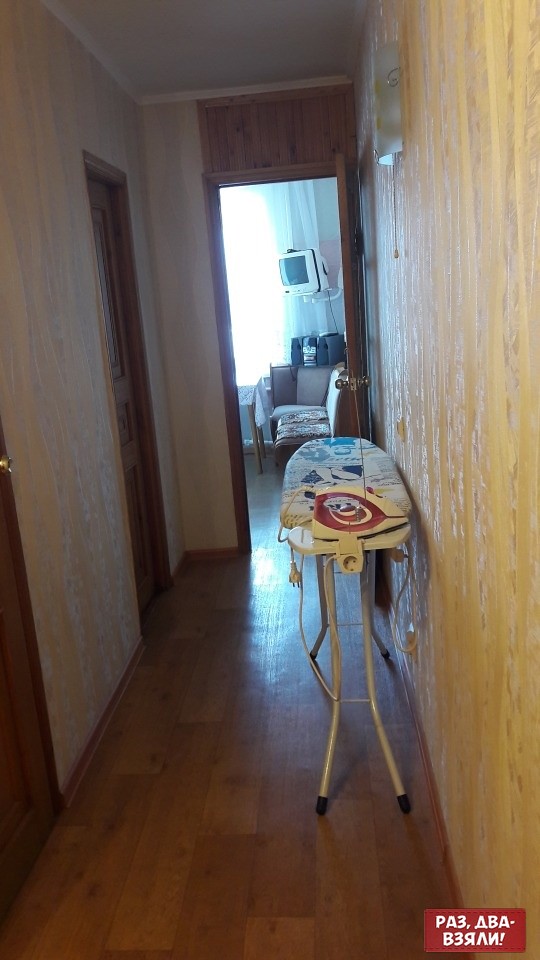This photograph captures a hallway inside a house characterized by its wooden hardwood flooring and walls with wood paneling. On the left side of the hallway, we see two closed brown wooden doors, while at the end of the hallway, there is a doorway leading to a brightly lit room. In the hallway stands an ironing board with metal legs and a fabric cover featuring black designs on a beige background. An iron is positioned at the edge of the board, with its cord hanging down. The walls of the hallway appear to be a yellowish-white or old beige color. Notably, there's writing in a foreign language ("PA3, ABA, B3RAN") at the bottom right of the image, displayed in white text on a reddish background. The room at the end of the hallway features a window with open curtains, through which light pours in, illuminating a light-colored chair and a wall-mounted white television.